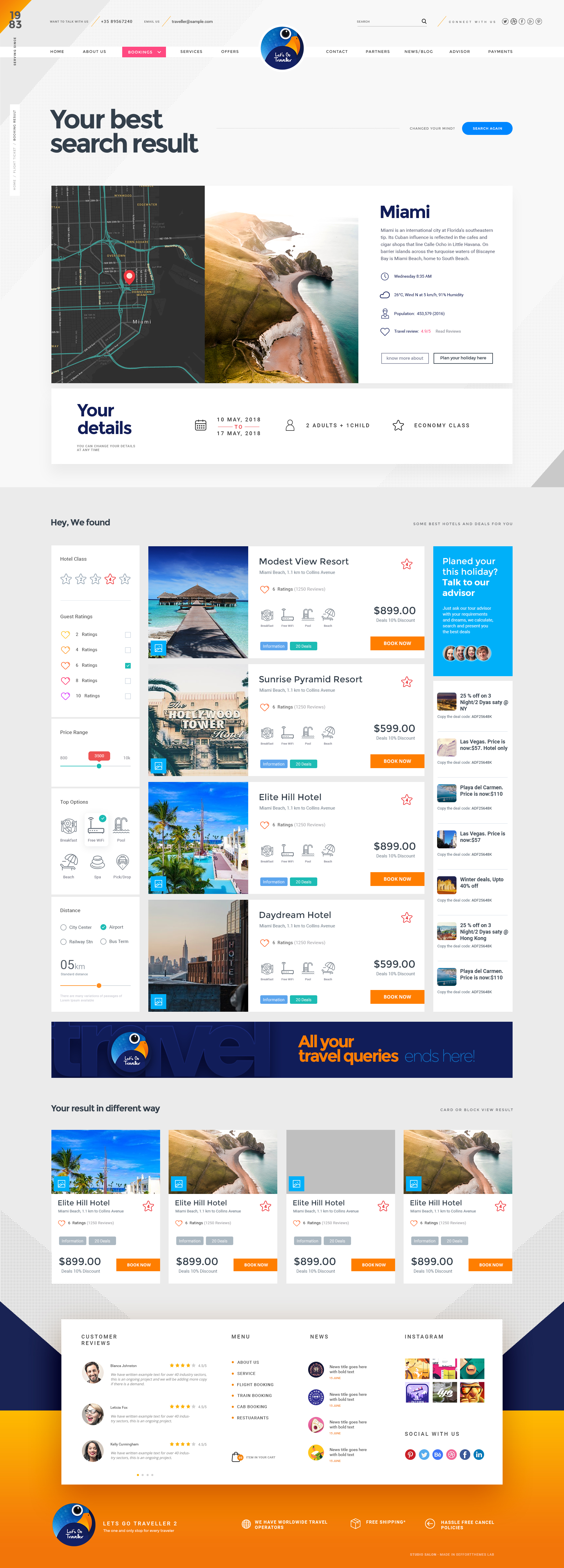This image is a vertical screenshot, likely taken from a webpage, presenting travel search results. The dimensions are roughly a 70:30 height-to-width ratio. The screen has a grayish background at the top with twisted text that reads "Your Best Search Results" on the left side. Below this, there is a circular logo of a blue bird with an orange beak and a black eye, outlined in white. Under the logo, there is a small segment of white text.

Further down, a white box with the word "Miami" is prominently displayed, accompanied by an image of a picturesque coastline. Below this image, there's a section showcasing various resorts in Miami, each represented with a thumbnail image and details. The resorts listed include "Modest View Resort" and "Elite Hill Hotel," both priced at $899, and "Sunrise Pyramid Resort" and "Daydream Hotel," both priced at $599.

At the very bottom, a blue banner features the text "All your travel queries end here" with the same blue bird logo from the top, reinforcing a consistent theme throughout the webpage.